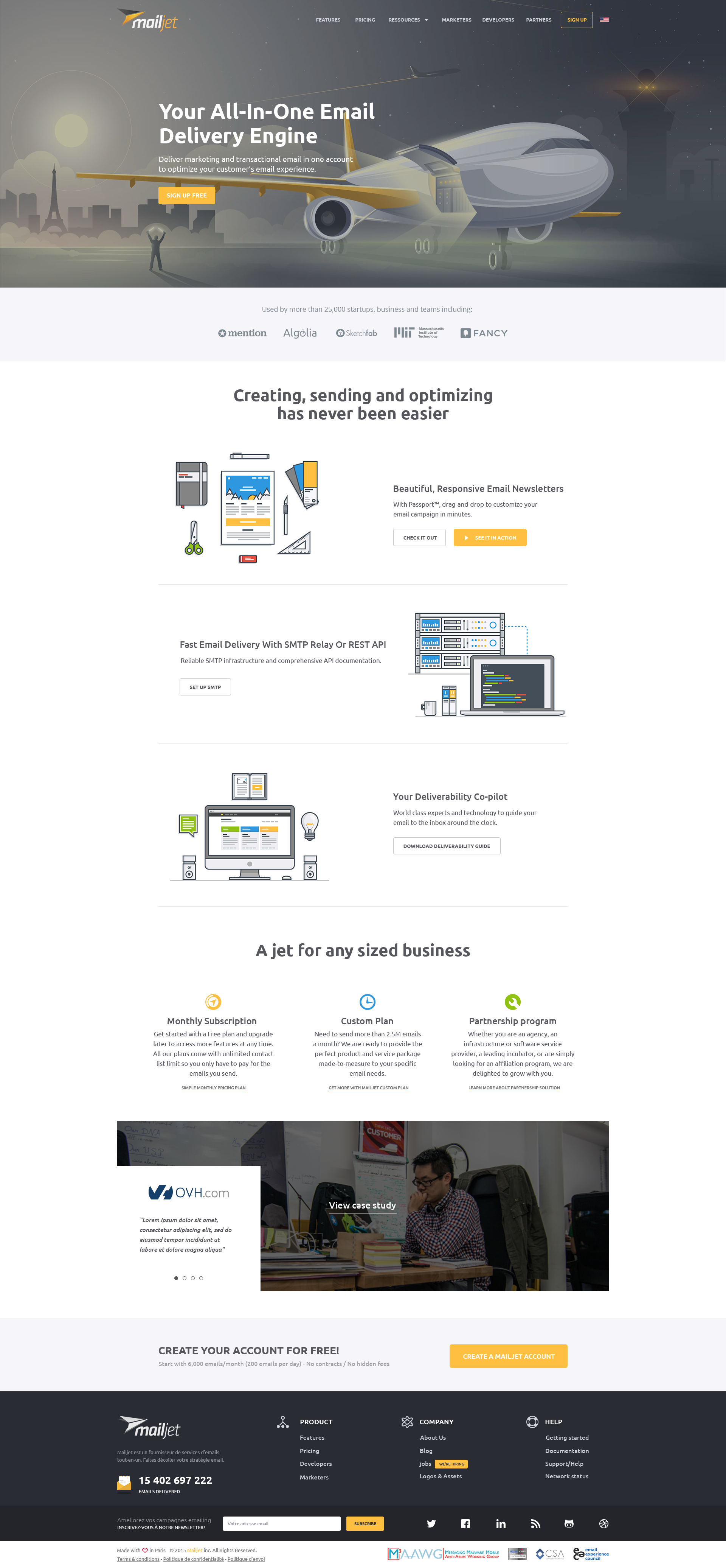Screenshot of the Mailjet Web Page: 

At the top of the screenshot, there is an artistic illustration featuring an airplane oriented to the right. The airplane is shaded in gray with distinctive yellow wings and is depicted stationed on a runway. To the left of the airplane, a human figure with raised hands is present. Adjacent to this scene, towards the left center of the section, there is a detailed drawing of the Eiffel Tower, adding a touch of Parisian flair.

Just below this illustration, a bold heading reads "Creating, sending, and optimizing has never been easier." Accompanying this text are various icons including documents, scissors, rulers, computers, and light bulbs, symbolizing the array of tools and features available.

In the center of the page, a prominent slogan states, "A jet for any sized business," emphasizing the versatility of the service. The web page is divided into three horizontal sections filled with additional information, highlighting different aspects of Mailjet's offerings.

At the bottom of the screenshot, another image features a man seated at a desk, facing to the left, suggesting a business work environment. This visual likely aims to connect with professional users and illustrate the practical application of Mailjet’s services.